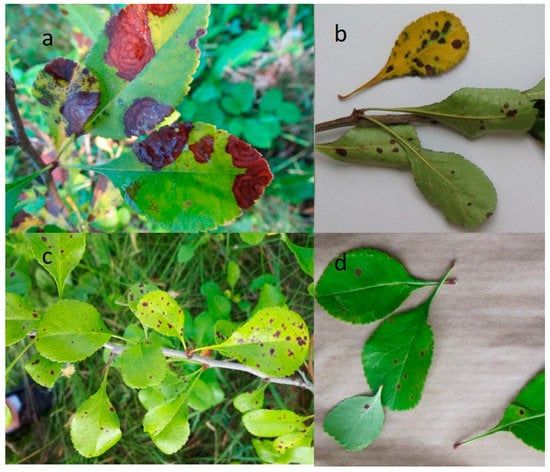The composite image showcases four rectangular sub-images (A, B, C, D), highlighting various stages and manifestations of leaf ailments on what appears to be leaves from the same plant species. 

- **Image A (Top Left):** This larger image displays a green, oval-shaped leaf with pointed tips, marred by thick, dark black and deep red patches that resemble burn marks, covering approximately 15-20% of the leaf's surface area.
- **Image B (Top Right):** A similar leaf specimen is presented on a countertop, exhibiting numerous smaller spots of the same black and red hues. This specimen is attached to a twig with several leaves, including a distinctly yellow leaf that is laying separate.
- **Image C (Bottom Left):** Another outdoor scene showing leaves on a plant, heavily dotted with smaller yet more numerous splotches compared to Image A.
- **Image D (Bottom Right):** Displays four leaves on a white background, with the same type of splotches but in a much sparser distribution; three leaves have a single dot, while the fourth has about five.

Overall, the images collectively emphasize the commonality of spotting and mottling across all the leaves, with significant variation in the size, number, and distribution of these spots.